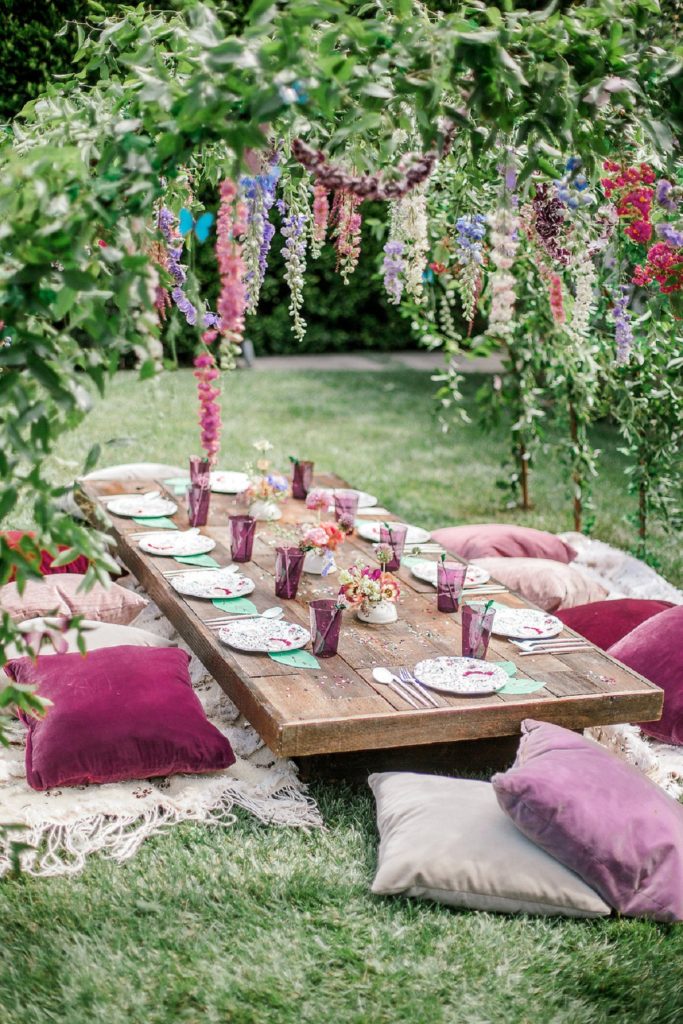The image depicts a charming outdoor celebration set up on a lush green lawn. A long, low wooden table, enough to accommodate ten place settings—four on each side and one at each end—serves as the centerpiece. The table is topped with elegant white plates featuring a subtle pink decorative design, along with silverware neatly arranged on the left side of each setting. Each setting also includes a distinctive purple glass. Three vibrant bouquets of multi-colored flowers grace the center of the table, adding a lively touch.

The seating arrangement consists of maroon, cream, pink, and red pillows placed on top of blankets spread across the grass, providing a cozy and laid-back atmosphere. An overhang of leaves and hanging flowers drapes above the table, casting a natural and enchanting canopy, perfect for a garden party. Capturing the serene daytime ambiance, the setting is ideal for a picturesque picnic or any celebratory event, elegantly blending comfort, style, and the beauty of nature.